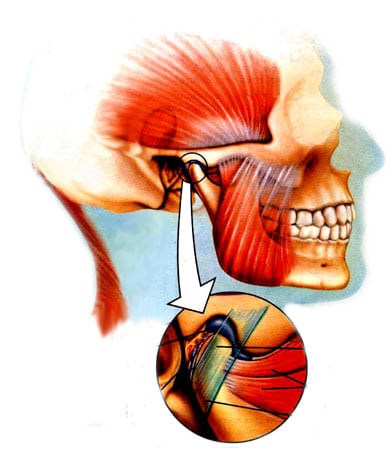This detailed educational image features a computer-generated illustration of a human skull, set against a white background with subtle blue accents. The focus is on the anatomical structure of the head, showcasing detailed depictions of the skull, jawline, and teeth. Red-colored muscles are illustrated in their anatomical positions, with white lines highlighting the muscle origins and insertions. The image provides a side view of the skull, elaborating on the jaw muscles and those located at the sides and back of the head.

Significantly, there is an emphasis on a specific area near the ear at the top of the jawline. This region is marked with a black circle and highlighted with a white arrow pointing towards it, leading to an enlarged view within a circular inset. This magnified section details a black bubble-like structure, indicating a notable feature or abnormality for educational purposes in the medical field. The intricacy of the diagram underscores its utility in studying and understanding human craniofacial anatomy.